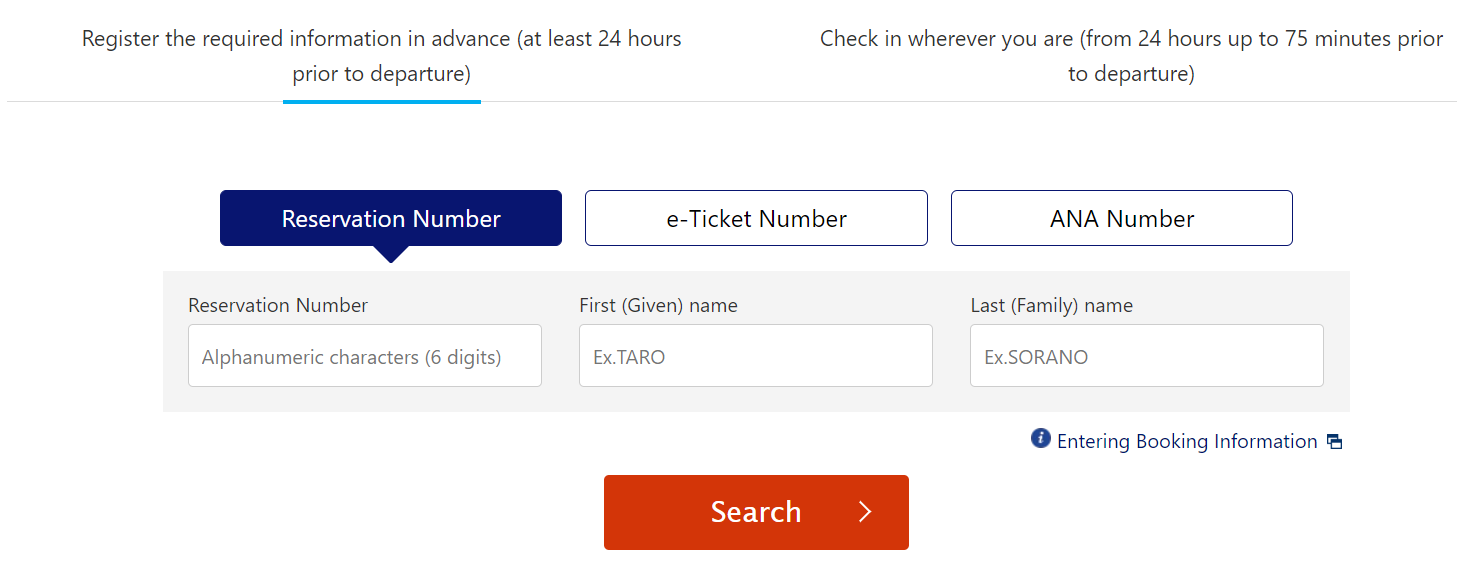This is a digital screenshot from an unspecified source displaying a user interface for registering travel information. The top section features a blue horizontal line underlining the directive, "Register the required information in advance, at least 24 hours prior to departure." To the right, it states, "Check in wherever you are from 24 hours up to 75 minutes prior to departure."

Below this directive are three rectangular selection options:
1. **Reservation Number** (currently selected)
2. **E-ticket Number**
3. **ANA Number**

Under the selected "Reservation Number," instructions read, "Reservation number: Alphanumeric characters, six digits," followed by fields to enter "First, given name (e.g., T-A-R-O)" and "Last, family name (e.g., S-O-R-A-N-O)."

At the bottom of the interface is a red rectangular button with the word "Search" in white letters.

The image is predominantly textual, lacks any photographic elements, and is wider than it is tall. There are no people, animals, birds, plants, flowers, trees, buildings, automobiles, or airplanes present in this image.